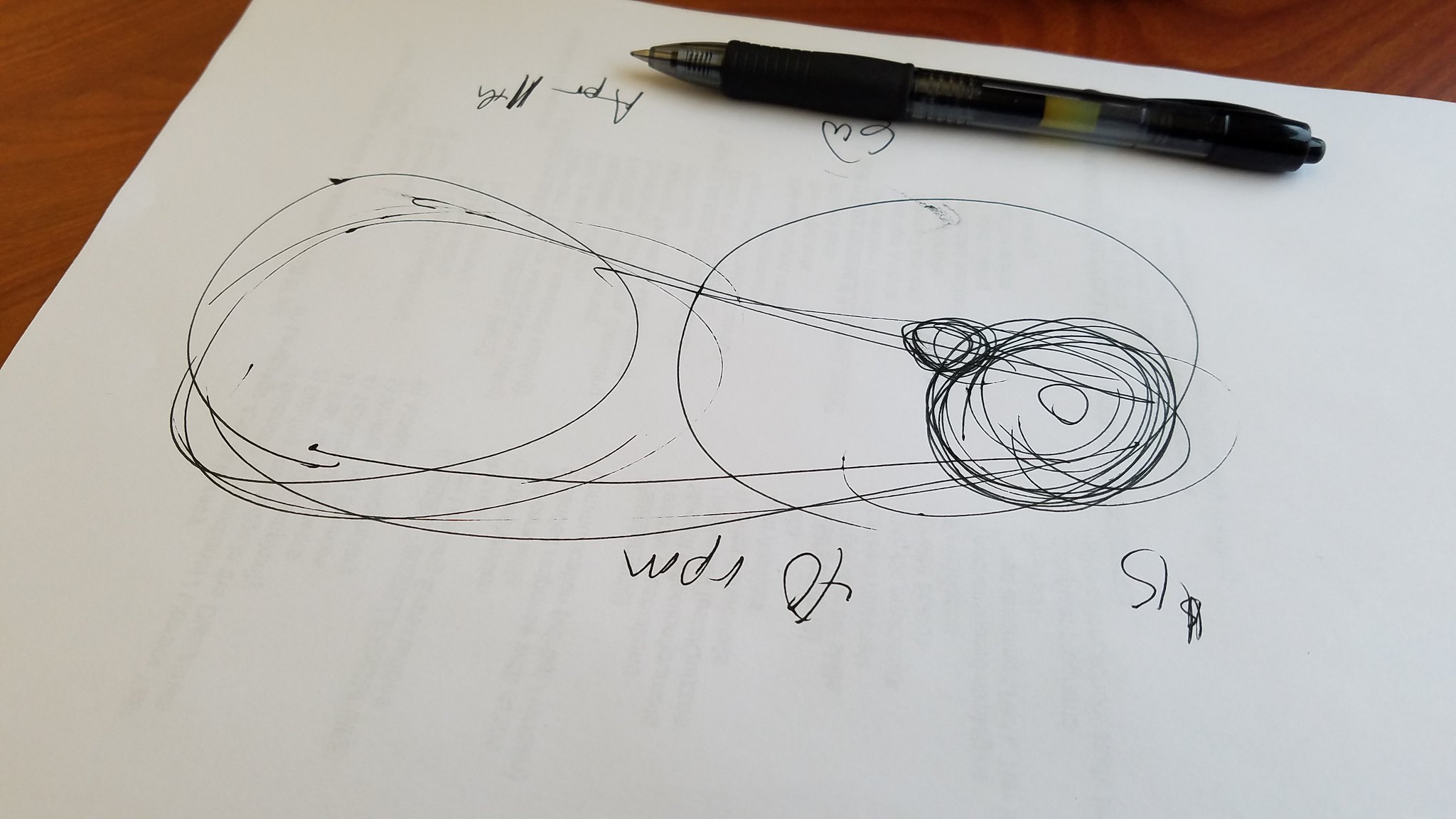The image captures a detailed drawing on a white piece of paper, set against a textured wooden surface, likely a table or floor. The wood, dark brown with visible grain patterns, lightens towards the left side of the photo, creating a natural gradient effect.

The drawing itself is centered, occupying about 90% of the frame. Prominently featured are two circles—a larger one on the right and a smaller one on the left. They are interconnected by looping lines resembling a chain linking two bicycle tires, suggesting motion or connectivity between the two circles. Additional scribbles and smaller circles surround the larger circle on the right, adding complexity to the diagram.

Annotations on the paper include "$15.40 RPM" positioned upside down above the large circle, indicating a specific rotational speed or rate, typically used in mechanical or scientific contexts.

A standard black ink pen lies diagonally across the paper, with the tip pointing left. The pen has a silver tip, a clear section where the tip emerges, a black grip, a clear barrel showing the ink level, and a black cap. Inside, the black ink is visibly followed by a yellow substance, a common feature in such pens designed to ensure smooth ink flow.

Overall, the photo is a well-composed shot capturing both the intricate drawing and the everyday object, the pen, providing a sense of scale and context.